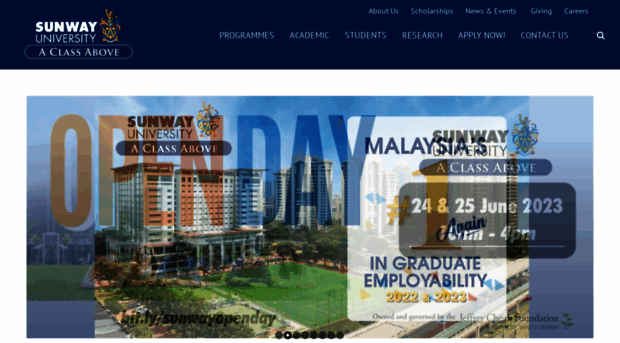This image showcases a promotional banner from Sunway University. At the top, a blue section prominently displays the university's branding. On the left, "Sunway" is written in bold white letters, with "University" directly below it in smaller white text. Below this, a bubble caption reads "A Class Above." To the right of the text, there is a distinctive logo resembling a peacock. Adjacent to the logo, a series of navigational tabs can be seen, labeled "Programs," "Academic," "Students," "Research," "Apply Now," and "Contact Us." Above these tabs, additional links include "About Us," "Scholarships," "News and Events," "Giving," and "Careers."

Below the navigational interface, the main imagery features a collage of faded images that come together to depict a large university building surrounded by a vast, green grassy area. Overlaid on this collage are labels and dates, culminating in the prominent text "Open Day," indicating an upcoming event or visitation opportunity at the university.